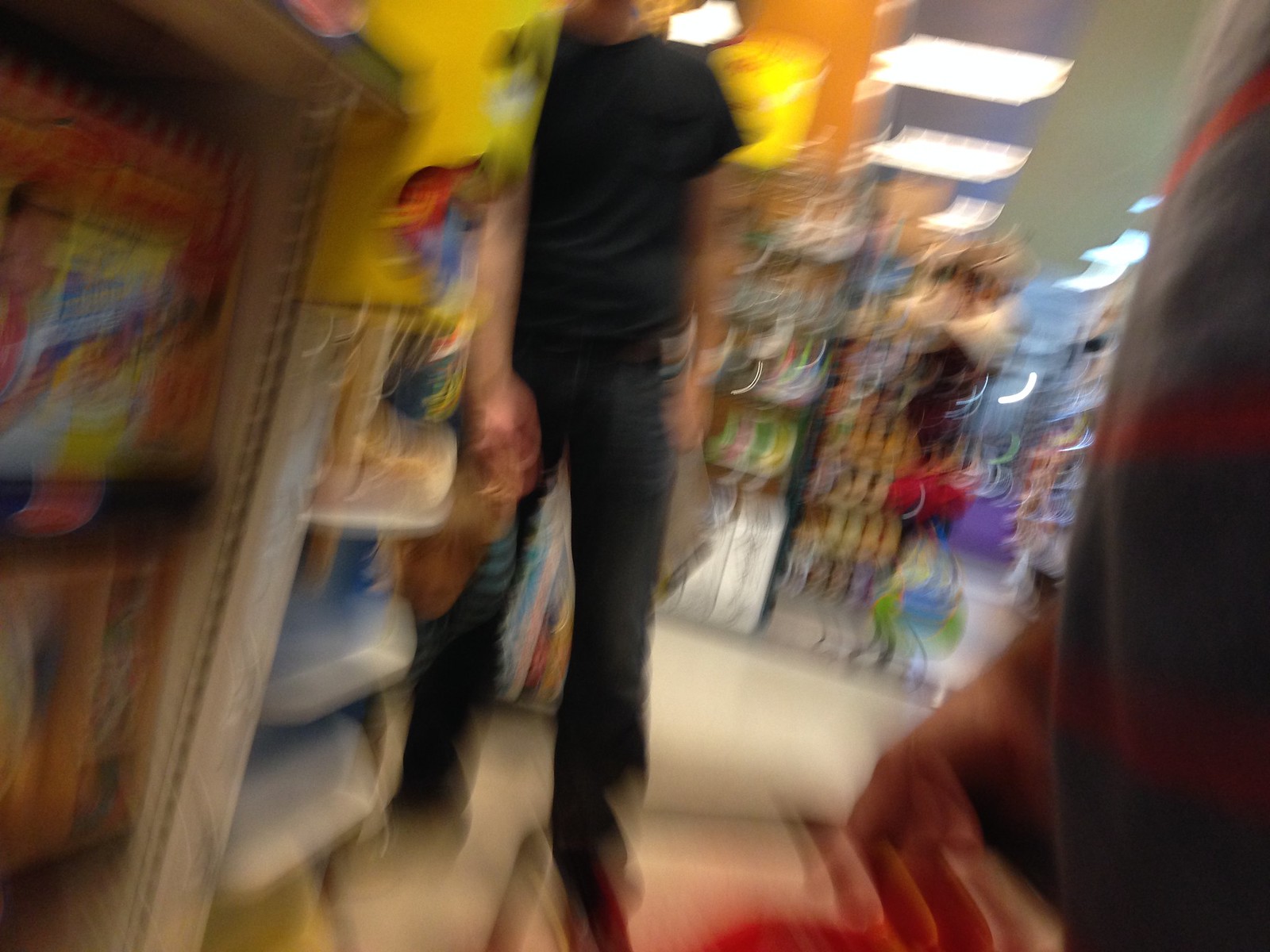This blurry photograph depicts the inside of a store with a slightly slanted angle to the right. Prominently on the left-hand side of the image, there are white shelves displaying bright colored merchandise. One notable item on these shelves is a yellow box, possibly cereal, featuring a character and a blue sash design. The floor of the store appears white.

In the middle ground, a person is visible, although their face cannot be seen. They are wearing a black short-sleeved shirt and dark jeans, and their hand, which is brown, is resting on a red shopping cart. There is also mention of another figure nearby wearing a gray shirt with red stripes, but details are less clear.

To the right of the image, there is a noticeable black object with red stripes, and a partially visible yellow display can be seen. Further in the background, the ceiling lights are rectangular and bright, illuminating additional merchandise hanging on pegs, primarily white and tan in color, towards the back of the store. The photo captures a bustling store aisle with a variety of items and displays, though the overall blurriness makes some details hard to distinguish.